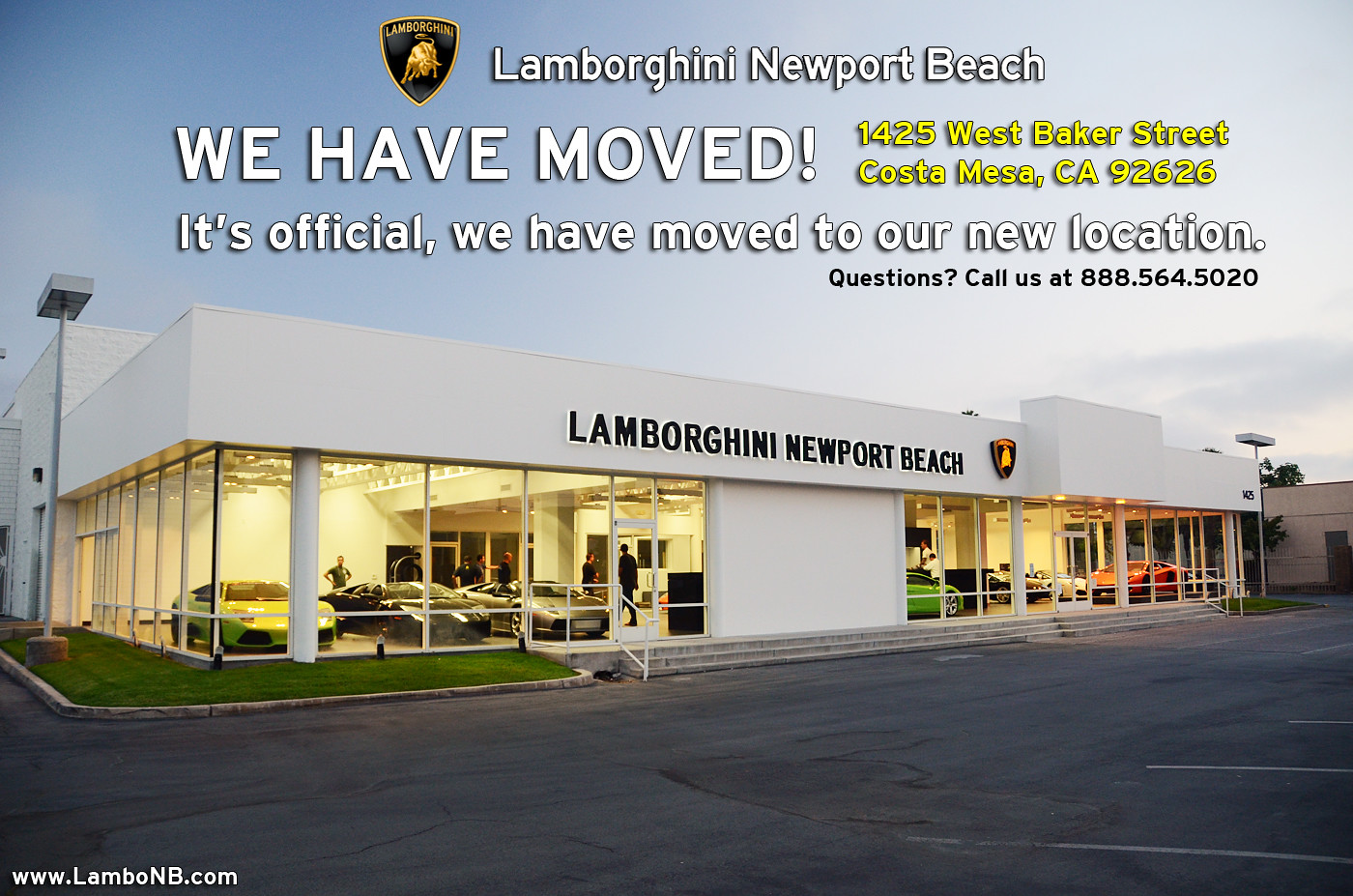The image is an informational announcement showcasing the new location of Lamborghini Newport Beach. The white, rectangular dealership building prominently displays "Lamborghini Newport Beach" in black lettering at the top. The structure features large glass panels with white frames, providing a clear view of the showroom filled with Lamborghinis in various colors. The entrance includes rectangular glass doors with white frames and a three-step concrete path leading to them. Multiple lines of text overlay the top of the image, reading: "Lamborghini Newport Beach. We have moved. 1425 West Baker Street, Costa Mesa, California 92626. It's official; we have moved to our new location. Questions? Call us at 888-564-5020." Additionally, the bottom left corner features the website: www.lambonb.com. The asphalt parking lot in front of the building has white lines demarcating parking spaces, and the building is brightly lit from within, contrasting with the dimmer exterior lighting.